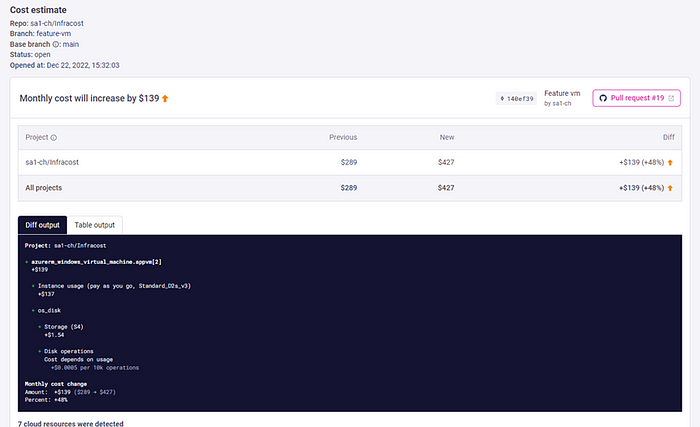The image displays a detailed software project page featuring a cost estimate report. The report includes several sections labeled as "Cost Estimate," "Repo," "Branch," "Base Branch," "Status," and "Opened at December 22nd, 2022." It indicates that the project's monthly cost will increase by $139. Prominently on the right side of the page, there is a pull request icon with the familiar GitHub logo. 

The content seems to involve infrastructure management as inferred from entries like "SA1-CH/infra-cost." The previous cost was $289, while the new estimated cost amounts to $427. Below these figures, there is a section displaying a "diff output," characterized by a black background with white text, presenting a detailed comparison of recent and previous project configurations. At the bottom of the page, a summary states, "Seven cloud resources were detected."

Overall, the image suggests a significant price hike in the services being used for software development, likely due to changes in infrastructure resource utilization.